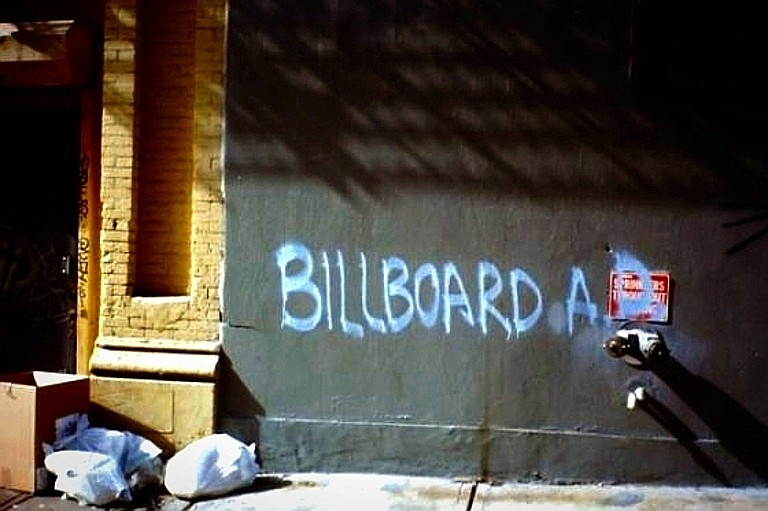The image captures an alleyway scene outside in a city street, featuring a close-up view of a building's facade. On the left side, a yellow limestone brick wall with a dark door is visible. Positioned in front of this brick wall, there is a two-foot-tall cardboard box and three white garbage bags. Adjacent to the brick wall, a larger black wall, spray-painted with the words "Billboard A.D." in white, dominates three-quarters of the image. The letter D in "Billboard" overlaps a red rectangular sign, possibly indicating a trespassing warning. Below the graffiti, a white fixture, potentially a hose hookup for firefighters, is partially visible. The scene is grounded by a simple gray concrete sidewalk that runs along the base of the walls, meeting the black painted surface on the right.